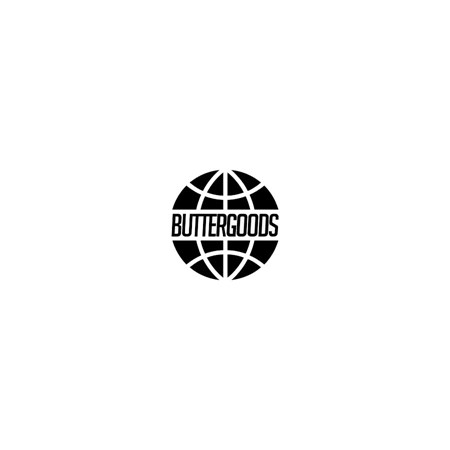The image features a professional, stylized logo set against a plain white background, prominently centered within the composition. It adopts a minimalist black-and-white color scheme. The logo resembles a simplistic, monochromatic representation of a basketball or perhaps a globe, emphasizing a sense of structure and balance. The circular emblem is intricately divided into 16 sections by lines that create triangular and trapezoidal shapes, mimicking the pattern found on a basketball. Prominently placed in the middle of this design is a white rectangle containing the text "BUTTER GOODS" in bold, black, all caps, sans-serif font. The lack of additional elements or text reinforces the focus on the logo itself, making it appear sophisticated and potentially associated with a brand related to sports or goods.